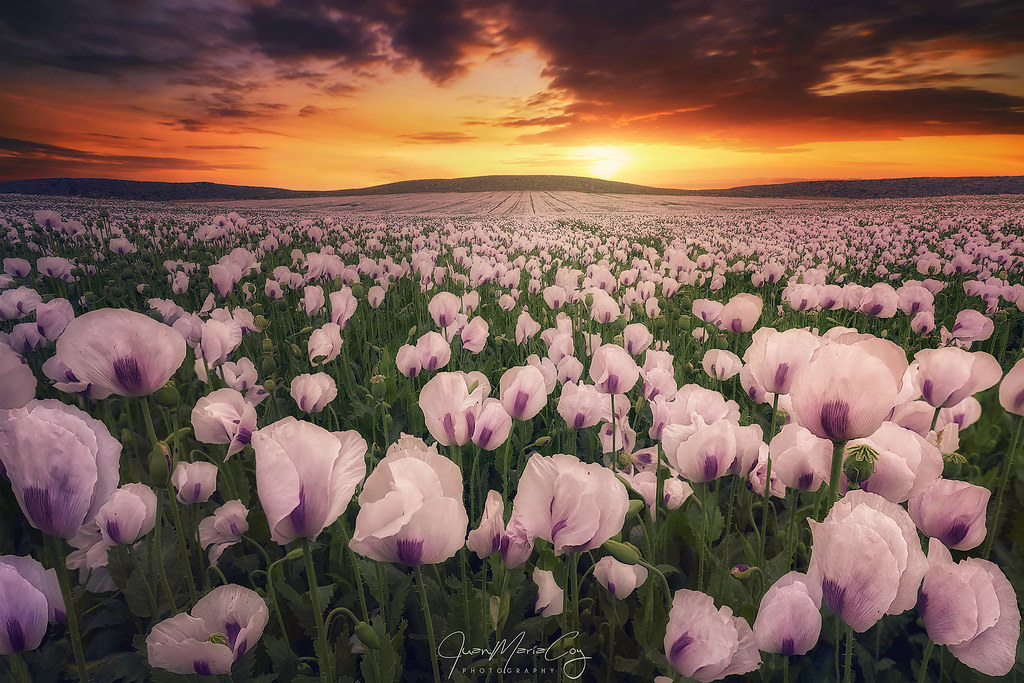The image depicts an expansive field of endless flowers that stretches from edge to edge and all the way to the horizon. The flowers, uniformly light pink with darker magenta centers, are perched on green stems with a hint of dark purple at the base. The scene is bathed in the warm hues of a vibrant sunset, with the sky displaying a fire orange color and dark clouds dotting the upper portion. The golden sun sits low on the horizon, casting golden rays across the field. In the background, rolling hills or distant mountains span the entire width of the image. At the bottom center, a white cursive signature of the photographer is visible, though accompanied by an illegible printed text.